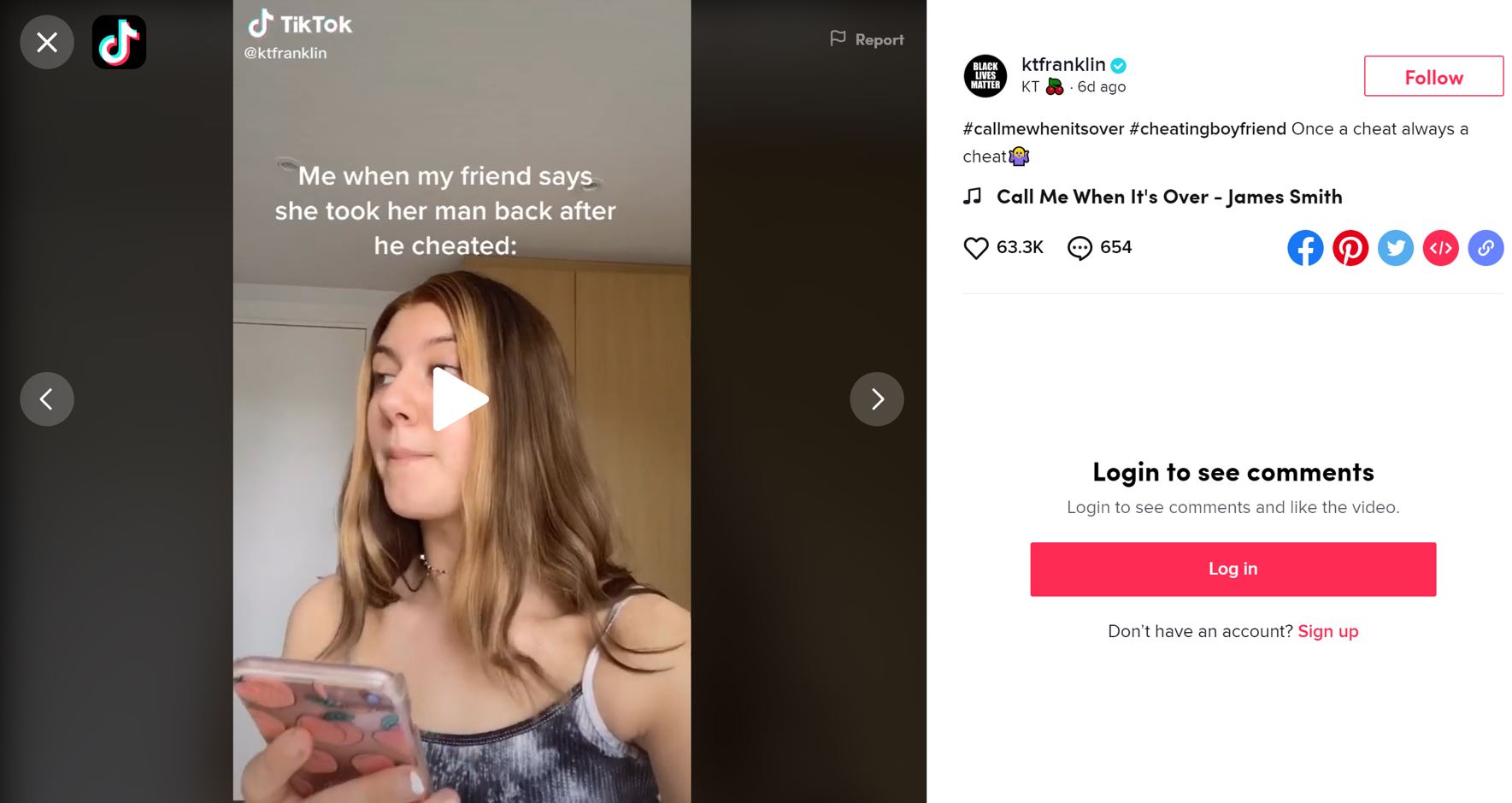A young woman, likely in her late teens or early twenties, is captured in the moment of about to play a TikTok video on her smartphone. The image features a TikTok interface where the video title reads, "Me when my friend says she took her man back after he cheated." The girl, adorned with a choker necklace, gazes slightly past the right, holding her phone with a peach-themed case in her right hand. The TikTok screen shows navigational options including an exit button, a report flag on the far right, and left-right swipe arrows. The video is flanked by two black vertical bars on either side.

In the background, a white door and a tall ceiling cabinet stretch from floor to ceiling. The TikTok video screen displays the username “ktfranklin” with the profile avatar and handle “@ktfranklin” in white at the top. It mentions “6 days ago” and features hashtags such as #callmewhenitsover, #cheatingboyfriend, and #once-a-cheat-always-a-cheat. A follow button is present, with the music titled "Call Me When It's Over" by James Smith playing in the background. The video has garnered 63,654 likes and numerous comments, though you must log in or sign up to interact using prominently displayed pink buttons at the bottom.